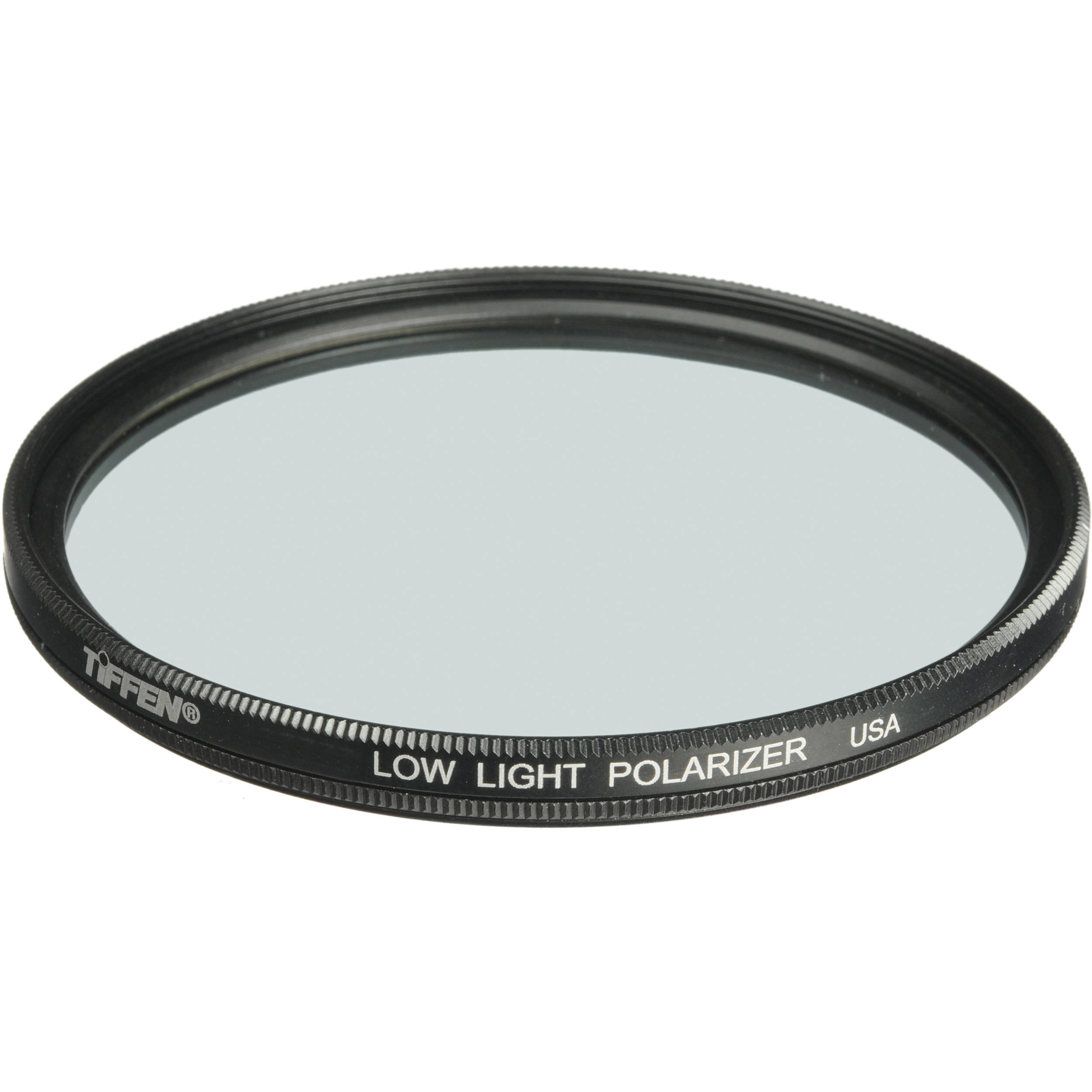The image features a black cylindrical lens with distinctive attributes. The rim of the lens, which is about one to two centimeters thick and covered with small zigzag ridges, contrasts sharply against the plain white background. The lens glass itself has a subtle grayish tint, adding to its sophisticated appearance. Prominently engraved on the side is the brand name "Tiffen," with the 'i' adorned by an unfilled diamond shape. This logo includes a registered trademark symbol (R). Centrally positioned and in bold white text are the words "LOW LIGHT POLARIZER," with "USA" slightly to the right. This type of lens, likely used for enhancing photography in dim lighting conditions, represents an older style for traditional cameras. However, the exact size of the lens remains indeterminate due to the lack of surrounding objects for scale.